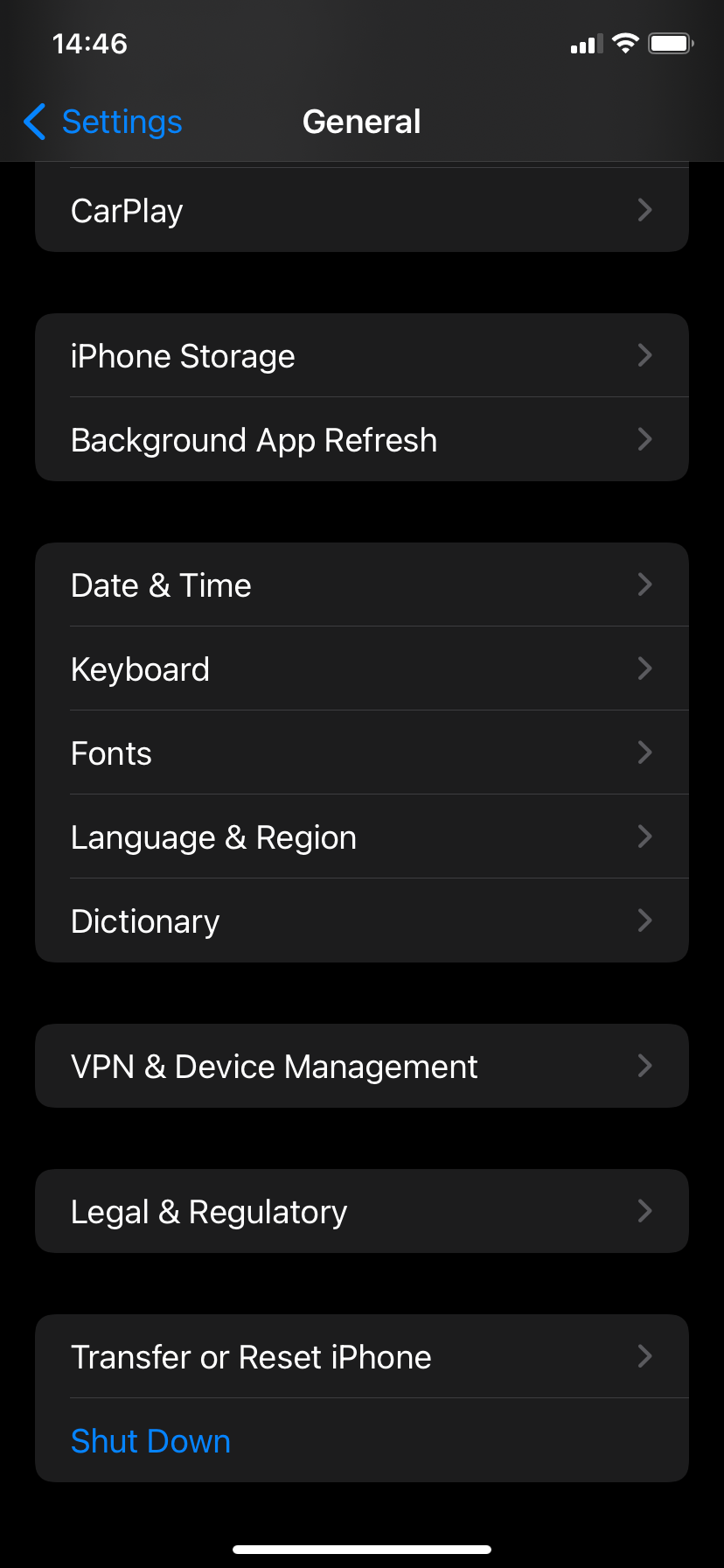The image is a screenshot of an iPhone's Settings menu. At the very top, the screen displays a navigation bar with the word "Settings" in blue text on the left side and a left-pointing arrow, both in blue. To the right of this, the word "General" appears in white text.

Below the navigation bar, the screen displays a series of options, each accompanied by a right-pointing arrow indicating further sub-menus. The outlined items and their arrangement are as follows:

1. CarPlay (appears to be at the bottom of a preceding section but partly cut off at the top of the image).
2. iPhone Storage and Background App Refresh are grouped together.
3. Date & Time, Keyboard, Fonts, Language & Region, and Dictionary are stacked together in a single section.

Further down, additional options include:
4. VPN & Device Management.
5. Legal & Regulatory.
6. Transfer or Reset iPhone.
7. At the very bottom, highlighted in blue text, is the "Shut Down" option.

The screen also shows a status bar at the top, with the time displaying as 14:46 in the top left-hand corner.